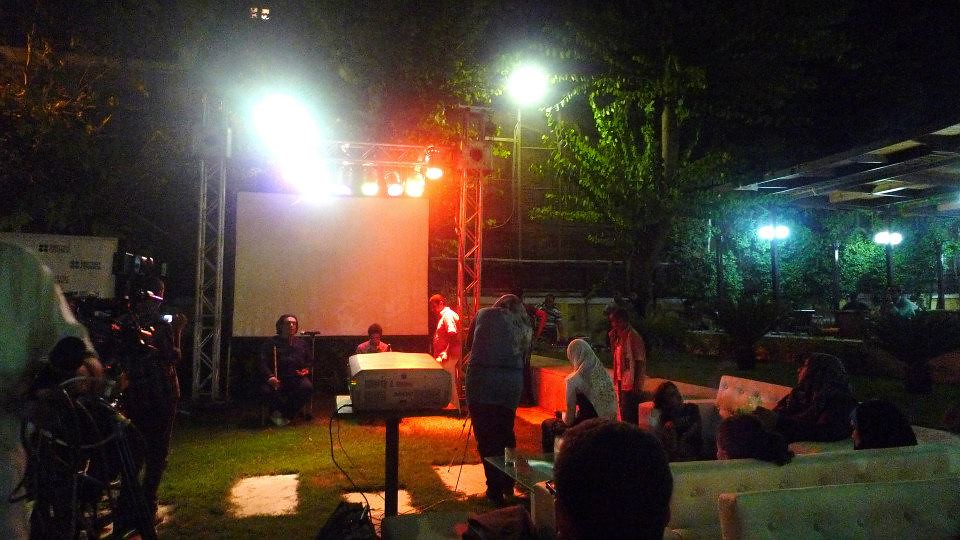The image captures an intimate, evening outdoor musical performance setup. Three gentlemen are getting ready to perform on a temporary stage, illuminated by multiple spotlights hanging from a steel cage above them. One of them holds a violin bow. They are positioned in front of a large projector screen, with the projector itself situated about 20 feet away in the center, operated by an individual either sitting or standing nearby. To the left side of the frame, there are cameras possibly from a local news channel, capturing the preparations. On the right side, a food court with people sitting at tables is visible, adding to the lively atmosphere. Close to the stage, a few couches and chairs are arranged in a square, where a small audience is seated, including a woman with a shawl and a man standing next to her. The setting suggests a night scene, likely held outside an event center, with additional smaller lights enhancing the ambiance.